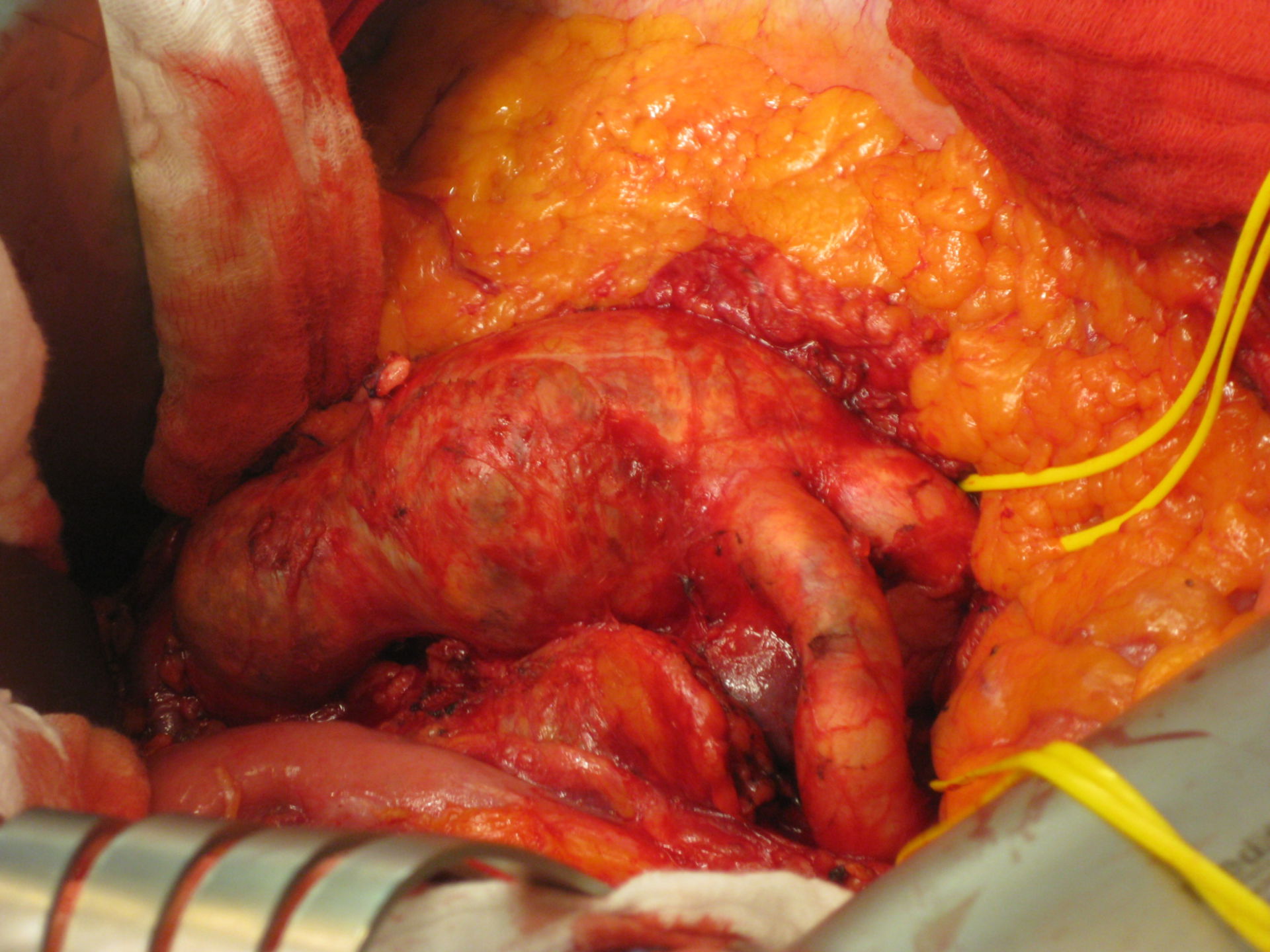The photographic image presents a detailed and close-up view of an indoor medical operation, showcasing various organs and surgical elements. The central focus is a red organ, possibly part of a heart or intestine, with visible blood on its surface. Adjacent to this is a squishy, orange component resembling fish roe or another section of an intestine. Attached to these are two distinctive yellow ribbons or tubes extending downward. The top left corner features white flesh, while the top right corner is dominated by a yellowish organ that extends downward. In the bottom corners, there are metallic surgical instruments; the left side includes a grooved metal piece, partially covered with red, while the right side shows more yellow ribbon material. Additionally, the bottom right corner includes a silver metal piece with brownish scratches alongside the yellow ribbons. Blood-soaked cloths or gauzes lie on the left side, further highlighting the surgical nature of the scene. The entire image is saturated with the wet, red appearance of exposed tissue, embodying the intense and visceral nature of surgery.